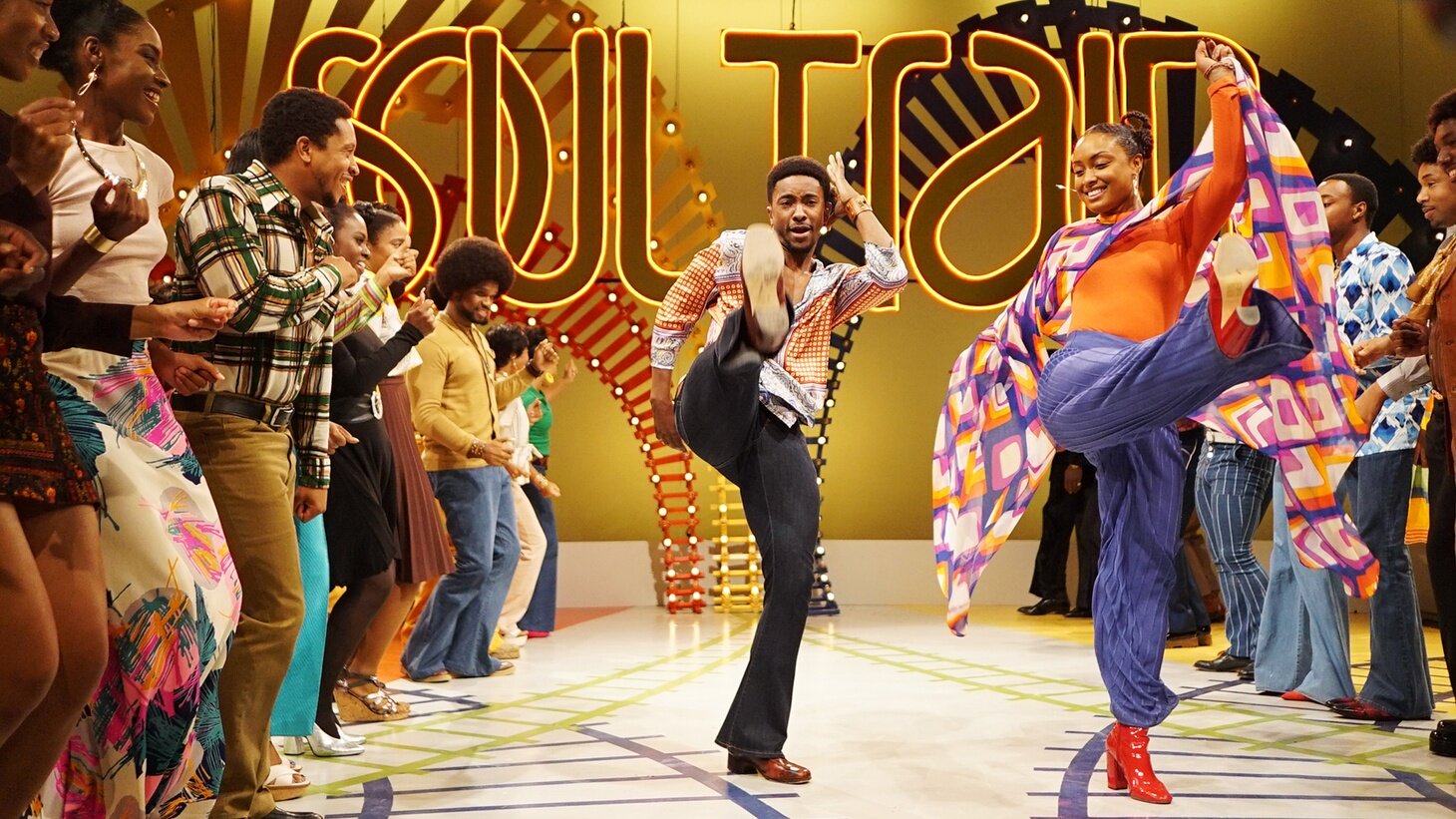This image is a lively snapshot from the 1970s television show, Soul Train, capturing a moment filled with vibrant colors and energetic dance moves. Against a gold-toned background, a large neon sign reads "Soul Train" in bright yellow letters, illuminating the scene. The foreground showcases a diverse group of young African-Americans lined up on both sides, observing two central dancers who steal the spotlight. The male dancer, sporting an orange-striped hoodie with gray pants and brown shoes, has one leg kicked up and his hand stylishly positioned near his light Afro. Beside him, a female dancer mirrors his pose, her red boots and blue pants complemented by an orange top and a colorful scarf flowing from her hand. The joyous atmosphere is palpable, with onlookers cheering and immersed in the festive, technicolor ambiance typical of the 70s era fashion, complete with bell-bottom pants and groovy hairstyles.